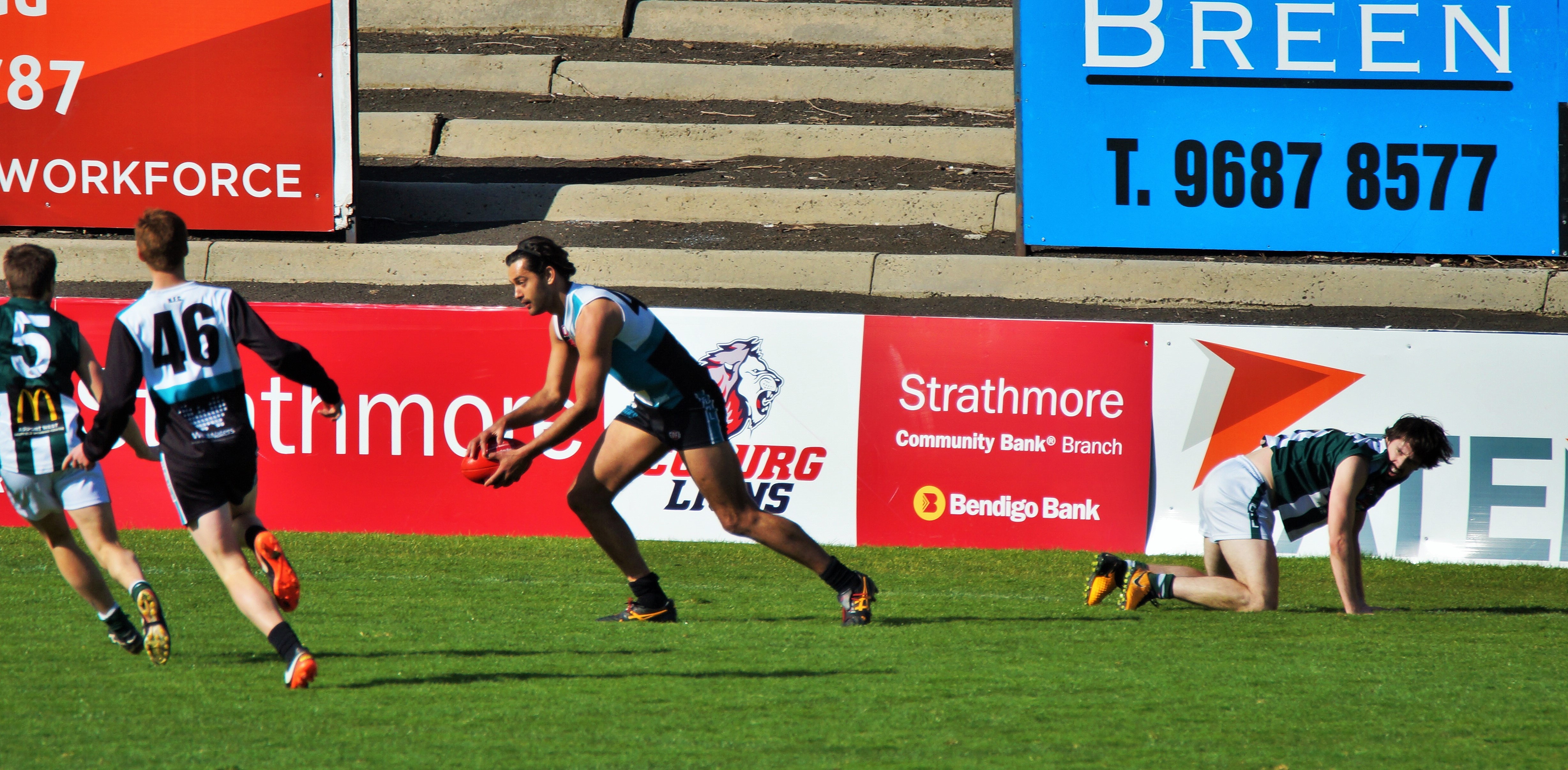In this image of a vibrant rugby game, set on a lush green field under open skies, four male players are at the center of the action. Clad in numbered jerseys and short shorts, the athletes are intensely engaged in the game. The player in the middle holds the oblong-shaped red ball, appearing poised to either pass or kick it, his body hunched forward in a dynamic motion that animates the scene. To his right, another player is down on all fours, seemingly recovering or strategizing his next move, while two players on the left are caught mid-stride, their legs and knees lifted as they sprint. The backdrop features a stone stadium with red, white, and blue banners, prominently advertising Strathmore Community Bank Branch and Bendigo Bank, alongside signs bearing words like "Lions," "Breen," and various phone numbers, adding to the atmosphere of local community enthusiasm and spirited competition.